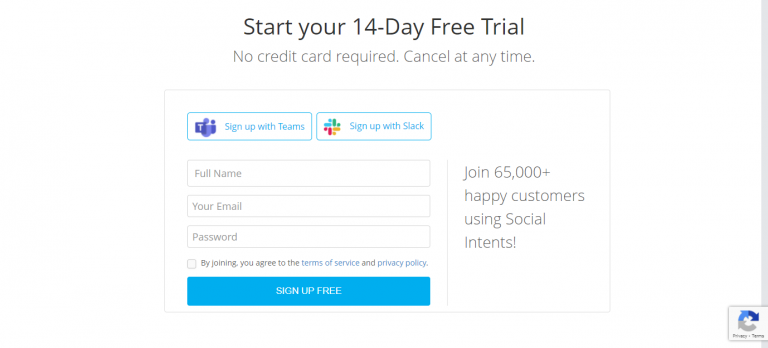Caption: 

A detailed view of a web app sign-up page offering a 14-day free trial without requiring a credit card and allowing cancellation at any time. The prominent message "Start your 14-day free trial, no credit card required, cancel at any time" is displayed in black and gray text on a white background. Beneath the offer, users can choose to sign up using either Microsoft Teams, represented by a purple "T" icon with a small people logo, or Slack, indicated by its colorful logo consisting of blue, green, yellow, and red elements. The form includes fields for entering a full name, email, and password, all of which are currently empty. There is an unchecked box beside a statement indicating that by joining, users agree to the terms of service and privacy policy. At the bottom, a blue button labeled "Sign Up Free" invites users to complete the sign-up process. The page highlights that over 65,000 customers are using the service, possibly named Social Intents, which integrates with Teams and Slack. The image is zoomed in, providing a clear view of the sign-up options and form.